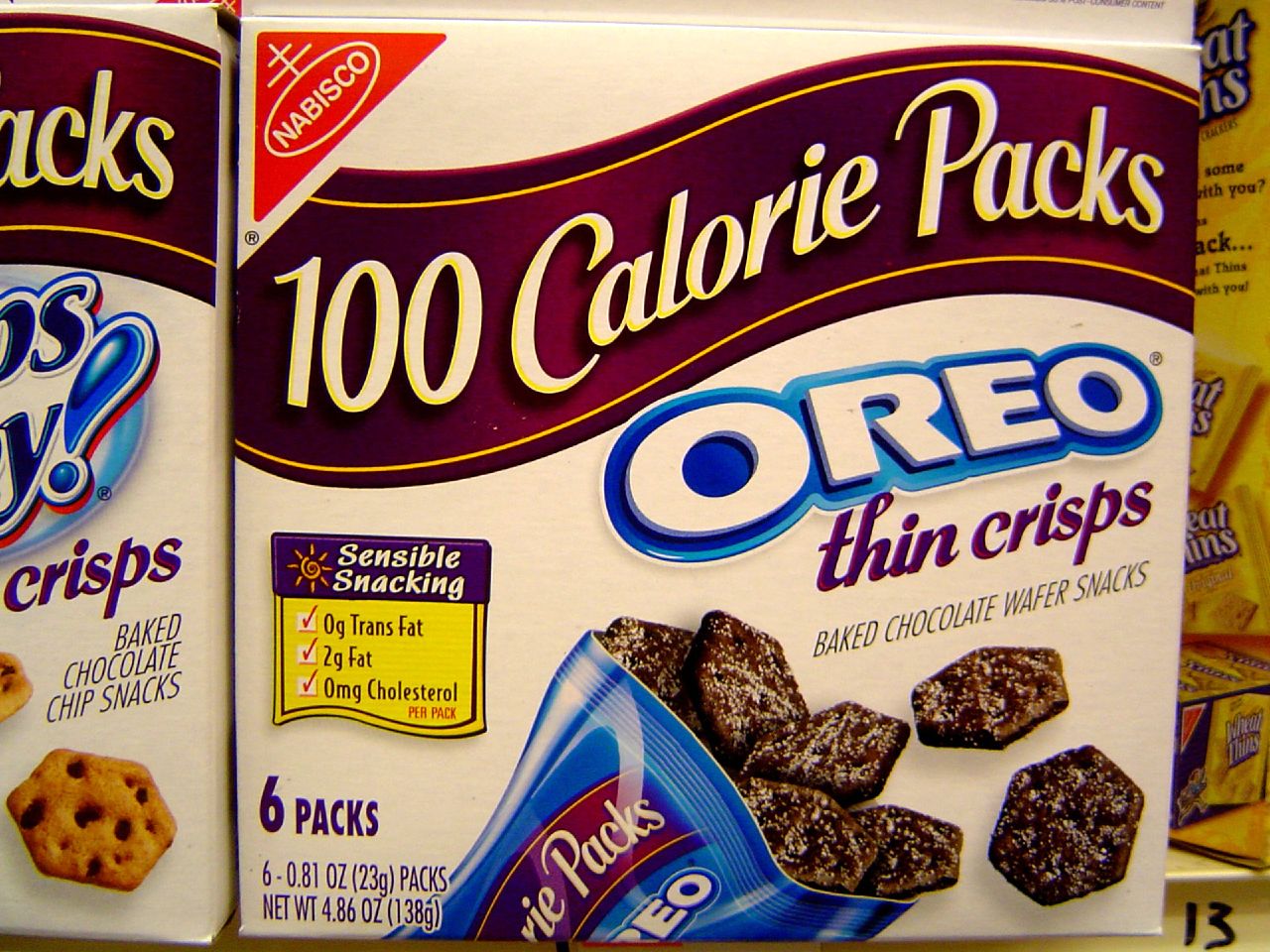This image features the packaging of Oreo Thin Crisps 100 Calorie Packs Snacks. The central focus is a white box with a red triangle in the upper left corner, indicating it as a Nabisco product. Across the top, a purple banner with yellow-lined edges prominently displays "100 Calorie Packs" in white lettering. Just below, the classic Oreo logo is visible, followed by "Thin Crisps" in a striking bluish-purple script. The phrase "Baked Chocolate Wafer Snacks" is elegantly printed in dark gray font beneath it.

To the left, a label declaring "Sensible Snacking" is positioned, accompanied by information highlighting its healthier nature. The packaging specifies there are 6 individual packs, each weighing 0.81 ounces. Centered on the box is a visual representation of the chocolate wafer snacks.

Adjacent to this box, a partial view of a similar packaging for "Chips Ahoy Crisps" is visible on the left side. In the background, there seems to be another snack, resembling a wheat thin. This comprehensive layout emphasizes the product's appeal as a convenient and healthy snacking option.